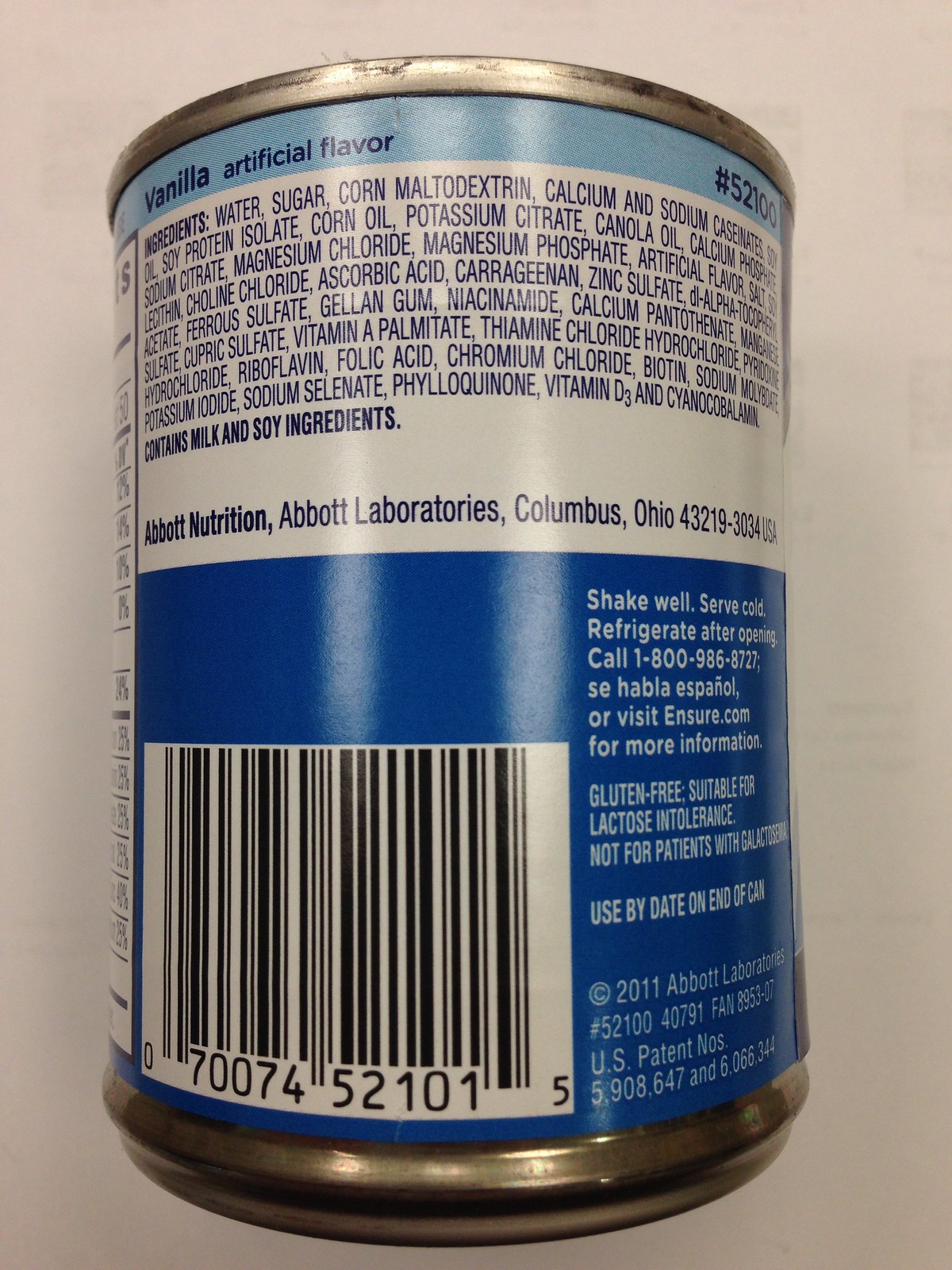The photograph depicts the back of an Ensure can set against a light gray to off-white background. The top of the can reveals the silver metal, and below it, the label transitions through shades of blue and white. Prominently displayed at the top in dark blue writing within a blue border are the words "Vanilla Artificial Flavor" alongside the number "52100." 

A white section follows which lists the numerous ingredients, including water, sugar, corn, maltodextrin, calcium, sodium, soy protein isolate, corn oil, potassium citrate, canola oil, calcium phosphate, sodium citrate, magnesium chloride, magnesium phosphate, artificial flavor, and salt. The can also notes that it contains milk and soy ingredients, produced by Abbott Nutrition, Abbott Laboratories, Columbus, Ohio 43219-30341 USA.

Lower on the label, there is a blue section containing a barcode and additional product numbers (70074-521-015 and 52100-40791). Instructions written in white advise consumers to "Shake well, Serve cold, Refrigerate after opening," and provide a contact number, "1-800-986-8727," mentioning that Spanish speakers are available ("Si Habla Espanol"). The website "Ensure.com" is provided for further information. Notably, the can is labeled as gluten-free and suitable for lactose intolerance, though not for certain patients. The can's use-by date and various patent numbers are also referenced.